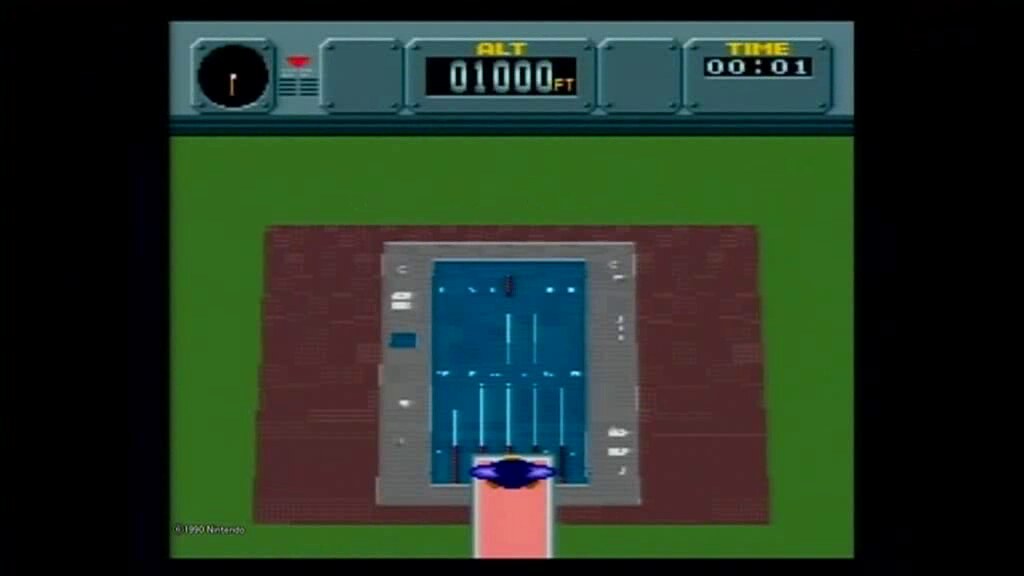The image resembles a video game interface set against a black background. Dominating the screen is a primarily green area, within which rests a purplish-red rectangle. Nested inside this rectangle is a smaller gray rectangle, and within that, a blue rectangle featuring two rows of vertical white lines.

Attached to this blue rectangle is a pink tab outlined in white, which bears an eye design with blue detailing. The inner blue rectangle appears to be the focal point where the game's action occurs.

At the top, there's a gray banner designed to mimic metallic compartments. On the left side of this banner is a black clock with a gold hand. Adjacent to it is another metal compartment displaying text in yellow letters. The main display reads "010000 feet" with a timer showing "1 second."